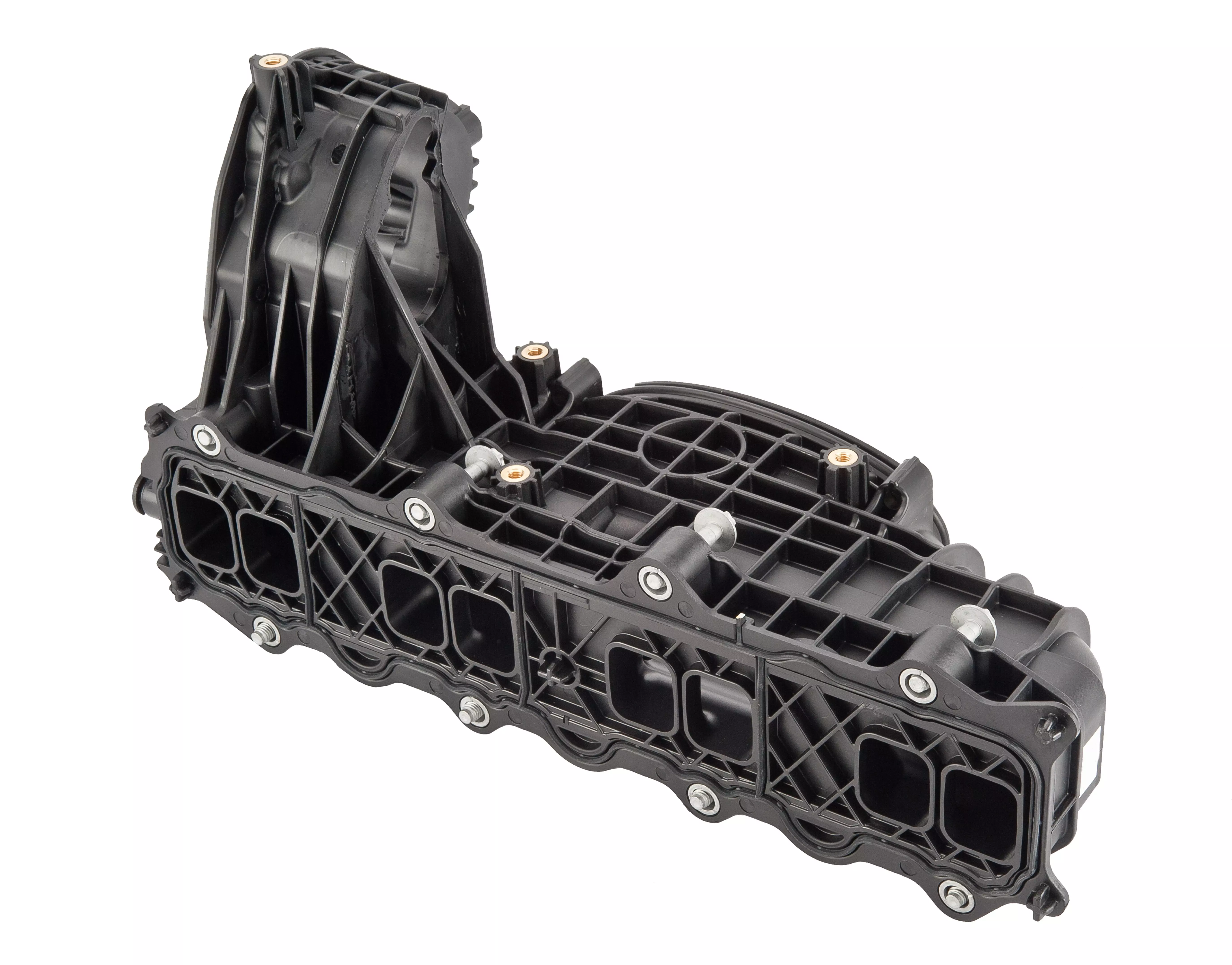This photograph depicts a vehicle's inlet manifold, meticulously crafted from black plastic and presented against a stark white backdrop. The manifold is prominently flat on both the top and bottom, with a notable rounded protrusion on its left side. The surface exhibits a detailed pattern with numerous silver screws or bolts embedded throughout, alongside golden-colored screw slots, offering a striking contrast. The object also features eight small, brownish-black sections, each shaped like a square and arranged in pairs, conducive to additional fixtures. The intricate criss-cross or grid-like design on the sides, reminiscent of a plastic crate, adds to its complexity. A gray, jagged gear-like structure can be observed protruding on the left side, contributing to the manifold's functional and aesthetic detailing. The entire piece appears in pristine condition, devoid of any noticeable damage.